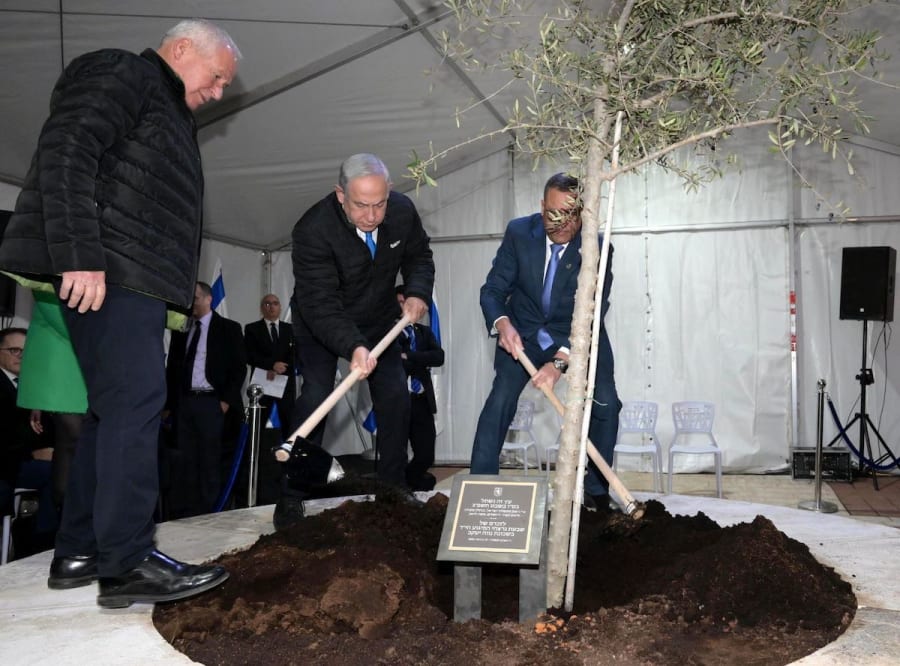In an outdoor setting beneath a large white, wedding-like tent, three men, all dressed in formal attire, are engaged in a tree planting ceremony. The scene features an older, light-skinned man with white hair wearing a fluffy black puffer jacket, black pants, and black shoes. He appears to be tapping his right shoe on the dug-up dark brown dirt. Beside him is a light-skinned man with gray hair in a black suit, white shirt, and light blue tie, who closely resembles Vladimir Putin. This man, bent over, is using a shovel to move the dirt. The third individual, partially obscured by the light tan tree trunk, is clad in a blue suit with a blue tie and black hair, also wielding a shovel to fill the hole around the tree. A plaque dedicated to the tree lies in front of it, though the inscription is unreadable. Surrounding them, the cream-colored tent shelters several other business people, all in suits, who are either conversing or seated on white chairs. Notable in the background are speakers set up on both sides, likely for facilitating speeches or audio during the ceremony.